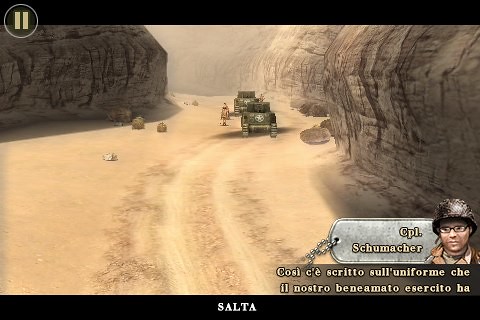This is a screenshot from a video game depicting a tense desert warfare scenario. In the foreground, the bottom of the screen displays the character Corporal Schumacher, with the name "Salter" written in what appears to be Spanish. The scene is set in a sandy area flanked by light, stratified rock faces, creating a naturally enclosed, perilous environment. Amidst this landscape, a couple of U.S. military vehicles, identifiable by the distinctive white star on a green background, are positioned, possibly with a soldier standing between them. The direction of their travel suggests they are moving through this rocky pass, heightening the sense of danger as they risk ambush. Despite the high-stakes atmosphere, the game's virtual nature ensures the consequences are contained to the digital world.